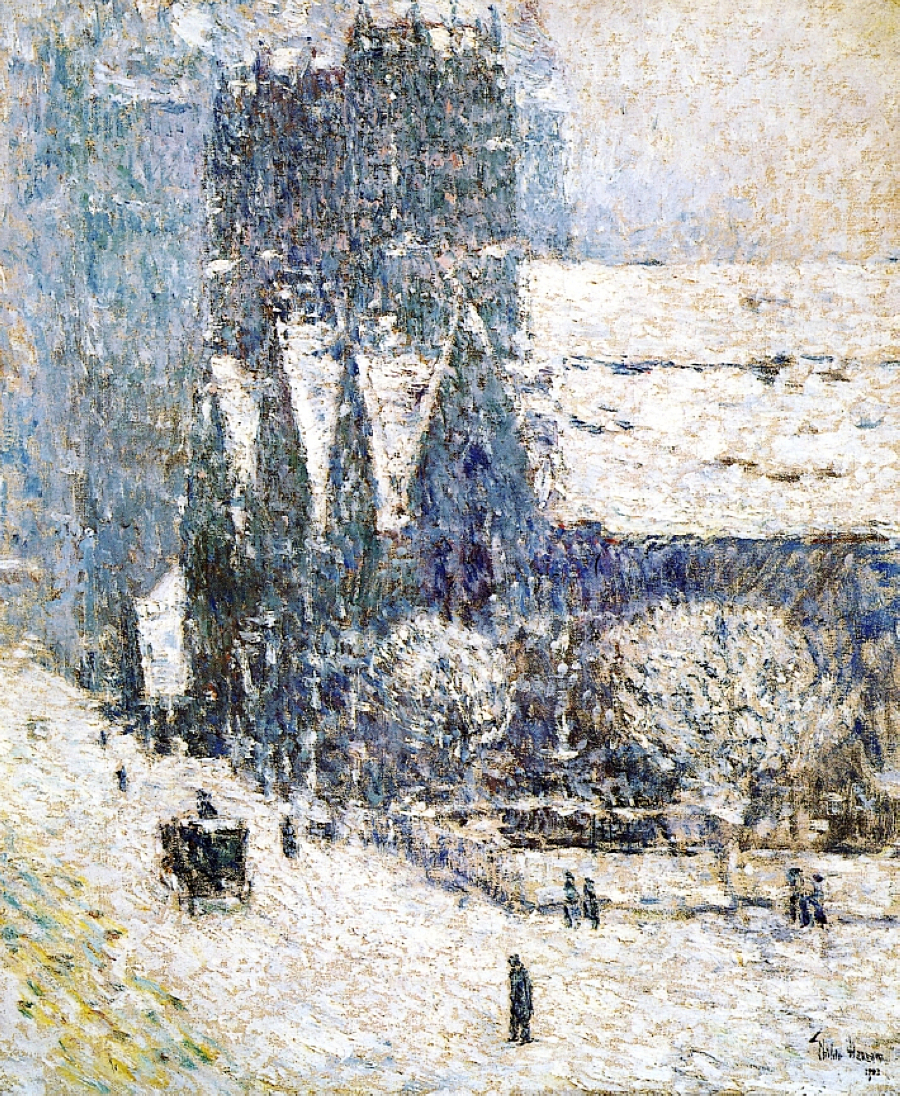This impressionistic oil painting, titled "Calvary Church in the Snow" by artist Hassam, depicts an outdoor winter scene in New York City during the daytime. The canvas showcases a large, majestic church with three distinct sections and blue towers rising into the sky. The structure is accentuated by white, snow-covered roofs and gabled sections, emphasizing the cold season.

In the foreground, three buildings with snowy gabled roofs stand prominently, blending into the snowy landscape. The scene captures a lively street corner where people, painted in shades of gray and black, walk alone or in pairs on the snow-covered road. A horse-drawn carriage, driven by a figure dressed in dark colors, moves towards the towering church. The cab's roof is laden with snow, exemplifying the wintry atmosphere.

Further adding to the scene's authenticity, trees sprinkled with snow frame the church, while the background transitions from a white upper right to a blue upper left, enhancing the ethereal quality of the sky. Near the bottom right corner of the painting, an inscription, though mostly illegible, appears to show the date "1782" and a signature.

Overall, the painting employs a palette dominated by grays and whites, with splashes of blue and other subtle colors, perfectly encapsulating the serene yet bustling ambiance of an old New York winter day.